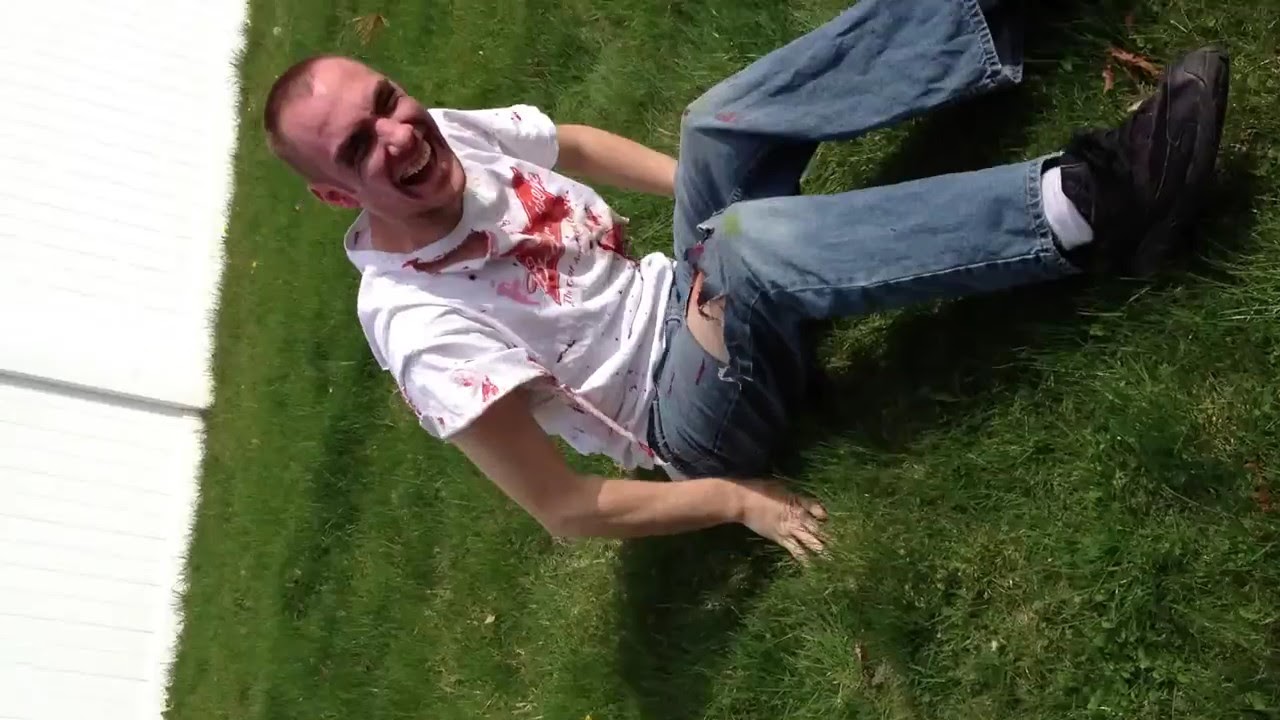In this detailed image, we see a man positioned at the center, sitting on a well-manicured grassy lawn. The shot is angled 90 degrees to the left. The man is wearing a short-sleeve white t-shirt that appears ripped near the neckline and bears red stains that might be paint or blood, with a recognizable Budweiser logo on the front. His blue jeans are torn above the knee on the right leg, and he pairs this with white socks and black shoes. He sports a short-cropped haircut with slight balding on the top, except for a small peak of hair in the center. The man is laughing heartily, showing his top row of teeth. His hands rest on the grass, with the grass covering about half the length of his fingers. On the left side of the image, which appears overexposed, there is a glimpse of a white vinyl fence. The setting suggests an outdoor, mid-day scene, likely in a backyard. The colors in the image include shades of white, gray, green, tan, blue, red, and pink, creating a vivid and detailed snapshot of the moment.